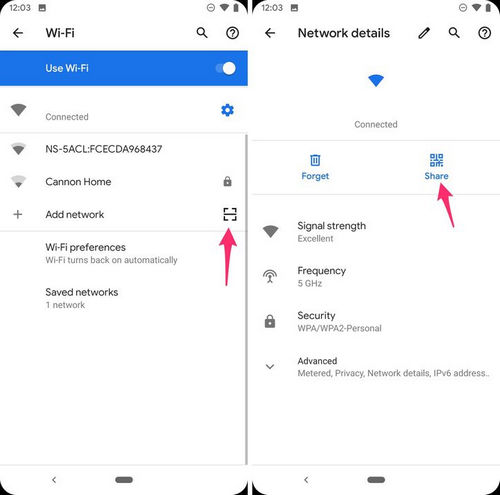The image displays two side-by-side screenshots of smartphone screens, showcasing different settings within the Wi-Fi menu. Both screenshots share identical top notifications: the top left shows the time as 12:03 with a small black square icon, and the top right includes a minus sign inside a circle, full Wi-Fi signal, and full battery indicator.

**Left Screenshot:**

- **Top of the Screen:** A left arrow labeled "Wi-Fi" against a white background, with search and question mark icons on the right.
- **Wi-Fi Settings Menu:** A prominent blue rectangle displaying "Use Wi-Fi" in white text.
- **Available Networks:** A list of several Wi-Fi connections. The top connection reads "Connected," followed by two other networks.
- **Additional Options:** Below the network list is a "+ Add network" option and a button with a square border. A red rectangle highlights this button.
- **Footer:** Options labeled "Wi-Fi preferences" and "Save networks."

**Right Screenshot:**

- **Top of the Screen:** The heading reads "Network details."
- **Wi-Fi Status:** A blue Wi-Fi signal icon is displayed in the upper-middle section with "Connected" below it.
- **Manage Network:** Two blue icons are present—a trash can labeled "Forget" on the left and a QR code labeled "Share" on the right, highlighted by a red arrow.
- **Additional Details:** Information on signal strength, frequency, security, and advanced settings is shown beneath the icons.
  
This detailed comparison clearly outlines the functionalities available within the Wi-Fi settings on a smartphone.